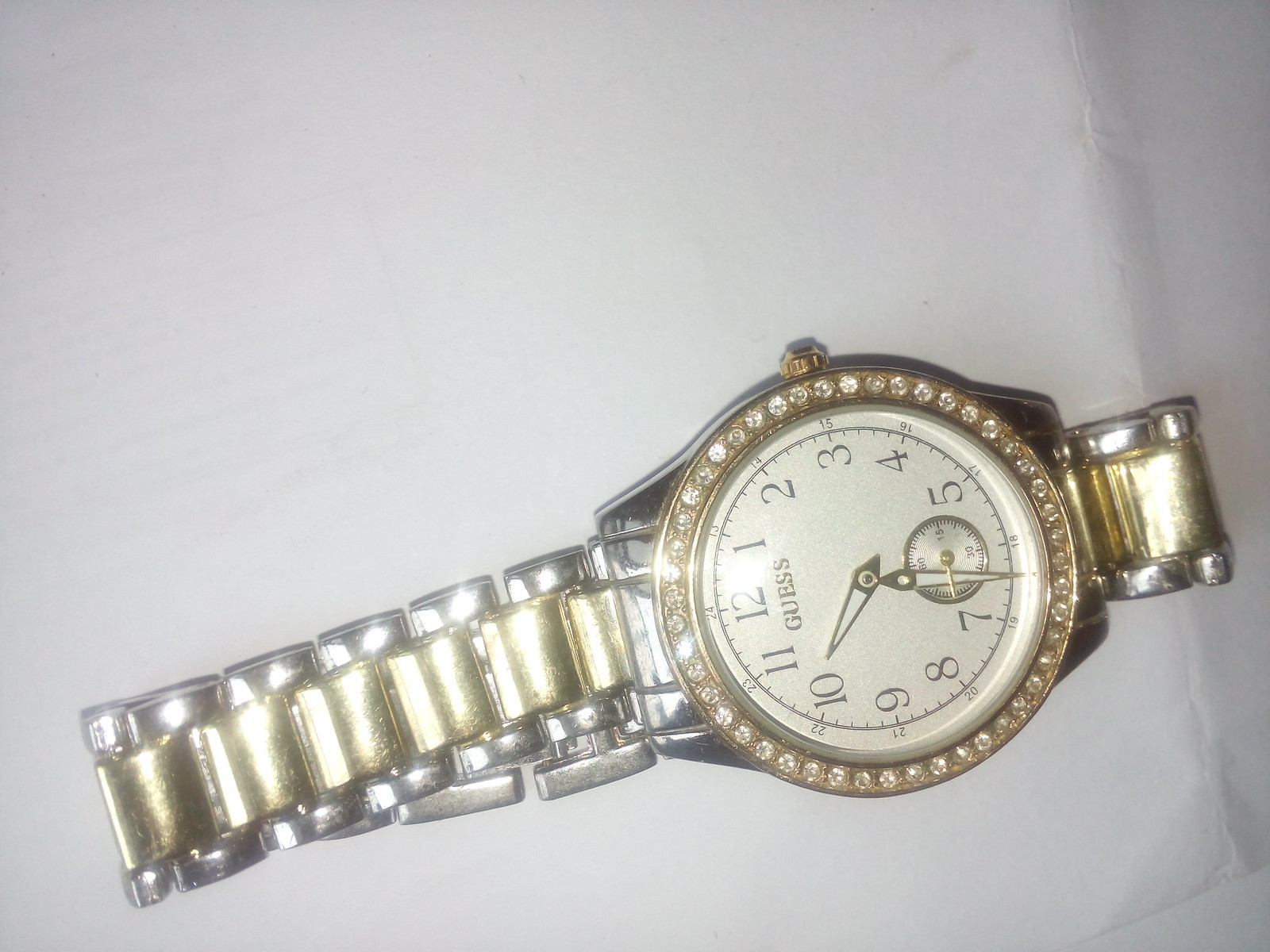This photograph captures a luxurious wristwatch elegantly displayed atop a white surface that appears to be a piece of folded paper or possibly a notebook. The watch is positioned in such a way that the metal band extends from the lower left corner of the image to the middle right. The band itself is an exquisite combination of materials, featuring silver edges and a center section adorned with gold-colored metal links. 

The watch face dominates the lower right portion of the image, showcasing its round design with a golden edge encrusted with diamond studs that exude opulence. The face of the watch is a pristine white, marked with Arabic numerals around the edge. Notably, the number twelve is oriented towards the lower left of the image. The hour and minute hands are triangular in shape, bordered with either gold or silver, and filled with white centers, adding a sophisticated touch to the overall design. This detailed composition highlights the intricate craftsmanship of the timepiece against a simple yet elegant backdrop.